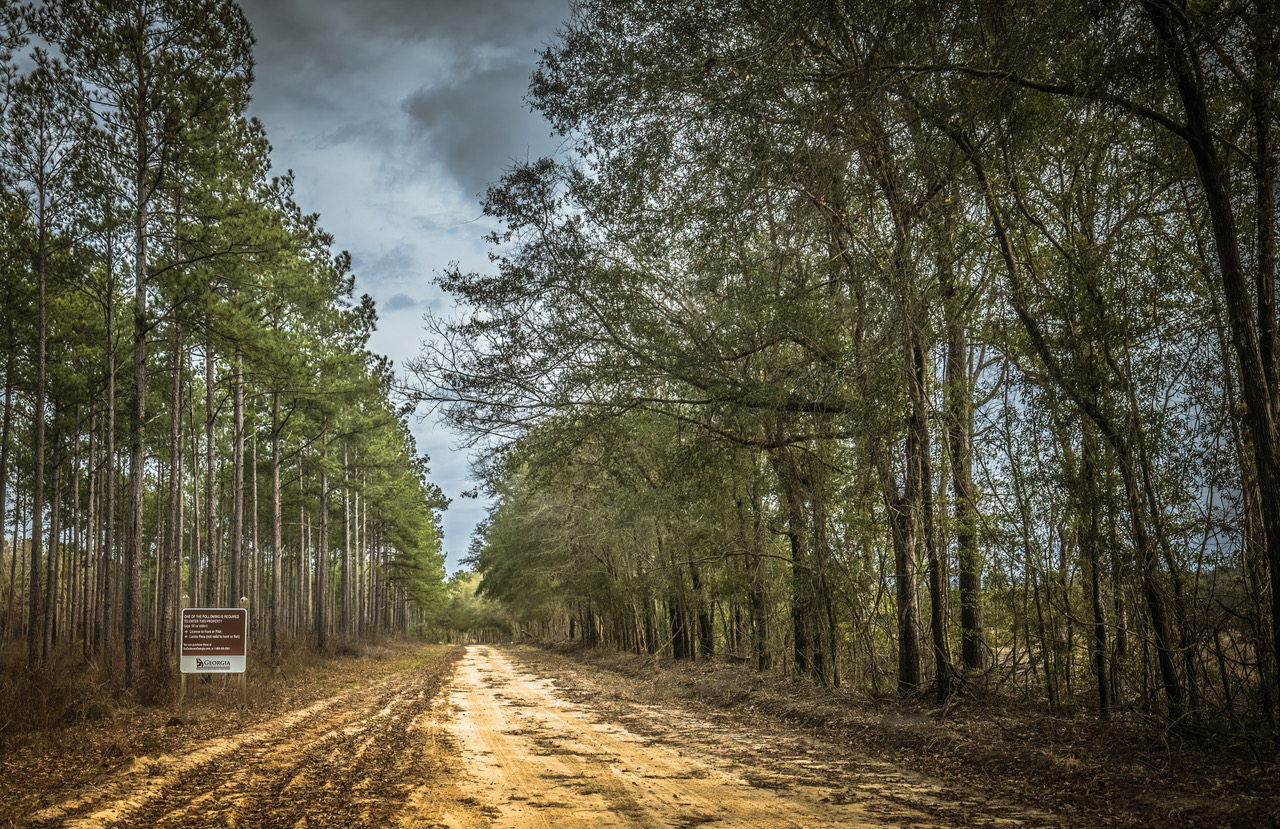A wide dirt road stretches into the distance, flanked by rows of tall, thin trees with varying degrees of foliage. On the left side, the trees appear to be uniformly planted, possibly man-made, with brown stems and trimmed tops, while the right side features more naturally grown trees, fuller with green leaves and brown branches. The road, a mix of beige sand, brown, and black dirt, displays scattered debris like twigs and leaves. Tire tracks mark the path, suggesting recent travel. A brown sign with a white border, typical of those seen at the entrance of nature preserves, stands on the left, though the text is too small to read. Above, the sky is a bluish-gray, filled with ominous gray and white clouds, hinting at an impending storm. In the background, rolling hills peek through the trees, contributing to the serene yet foreboding atmosphere of this natural setting.